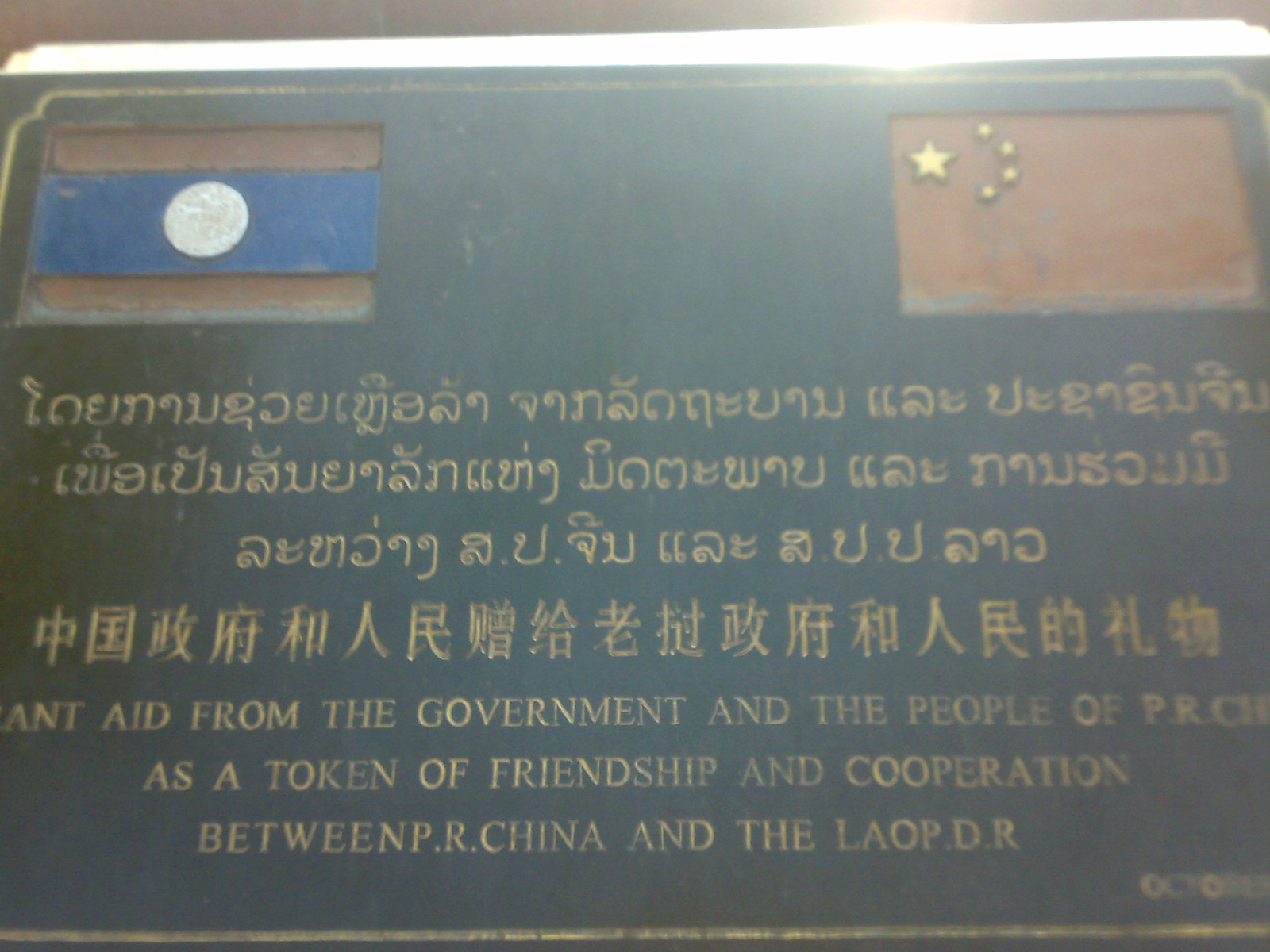The image depicts a close-up of a memorial plaque, likely photographed outdoors, with a visible beam of sunlight reflected at the top center. The plaque itself has a washed-out, dark green background with a thin, goldish-yellow border. At the top corners, there are two flags: the flag on the left is gray with a thick blue horizontal stripe in the center, featuring a white circle in its middle, while the flag on the right is the Chinese flag with a rusty red hue, showcasing one large star in the top left and four smaller stars in a semi-circle towards the right. Below these flags, there is text in three languages. The first language appears to be Central Asian, possibly Lao. The second set of characters seems to be Chinese. The third section, in English, reads: "Aid from the government and the people of PR China as a token of friendship and cooperation between PR China and the Lao PDR." The English text is written in a goldish font, completing the detailed elements of this ornate plaque.